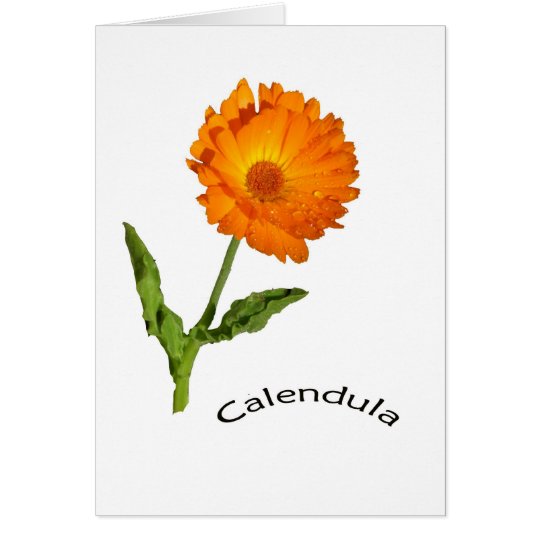This image depicts a greeting card displayed in portrait orientation, partially open so that only the front cover is visible. The card itself is off-white, creating a clean and simple background. On the front of the card, there is a striking orange and yellow calendula flower with an intricate circular center that is darker and accented with bright yellow highlights. The vibrant flower features multiple sets of petals, surrounding them are clear water drops that give a fresh appearance. This flower is perched on a green stem with two green leaves that are slightly curled, hinting at a natural, lifelike texture. Arched above the flower, the word "Calendula" is elegantly printed in black font. The inside of the card is not visible, leaving its contents a mystery, but the card does give the impression that it can be opened if desired.